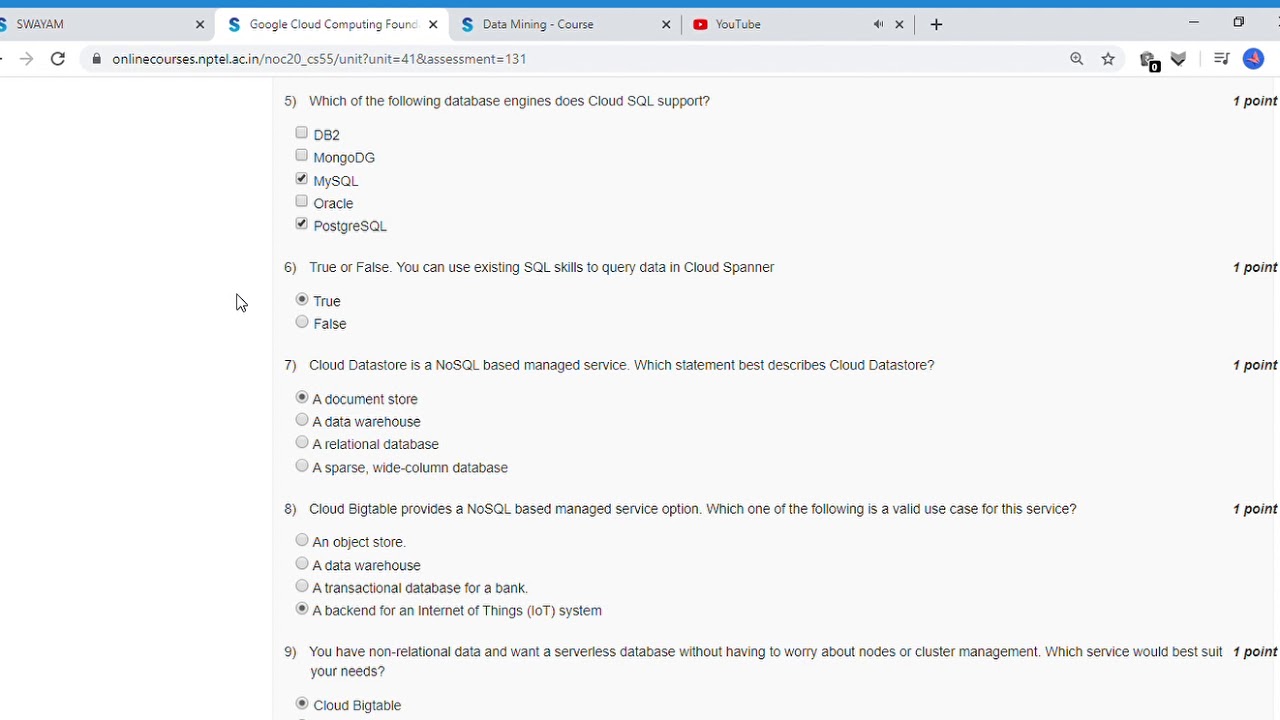The image is a screenshot taken from a computer, showcasing an online course platform with a predominantly white background and black text. Across the top of the screen, there's a light blue line, indicative of the browser's active tab section. Multiple tabs are open, including ones labeled "Swayam," "Google Cloud Computing Found," "Data Mining Course," and "YouTube." 

The URL in the address bar reads "onlinecourses.nptel.ac.in." Below the address bar, there are questions visible on the screen, arranged in a quiz format. The visible questions range from number five to number nine, each presenting a query related to cloud computing and its services.

Question 5 asks, "Which of the following database engines does Cloud SQL support?" The options selected are "MySQL" and "PostgreSQL.”

Question 6 is a true or false query stating, "You can use existing SQL skills to query data in Cloud Spanner," with "True" marked as the selected answer.

Question 7 reads, "Cloud Datastore is a NoSQL-based managed service. Which statement best describes Cloud Datastore?" The chosen response is "a document store."

Question 8 asks, "Cloud Bigtable provides a NoSQL-based managed service option. Which one of the following is a valid use case for this service?" The answer clicked is "a backend for an Internet of Things (IoT) system."

Question 9 presents, "You have non-relational data and want a serverless database without having to worry about nodes or cluster management. Which service would best suit your needs?" The selected option is "Cloud Bigtable."

Adjacent to each question on the right side, there are indications of points, with each question marked as "1 point," suggesting either the scoring per correct answer or the total points available per question.